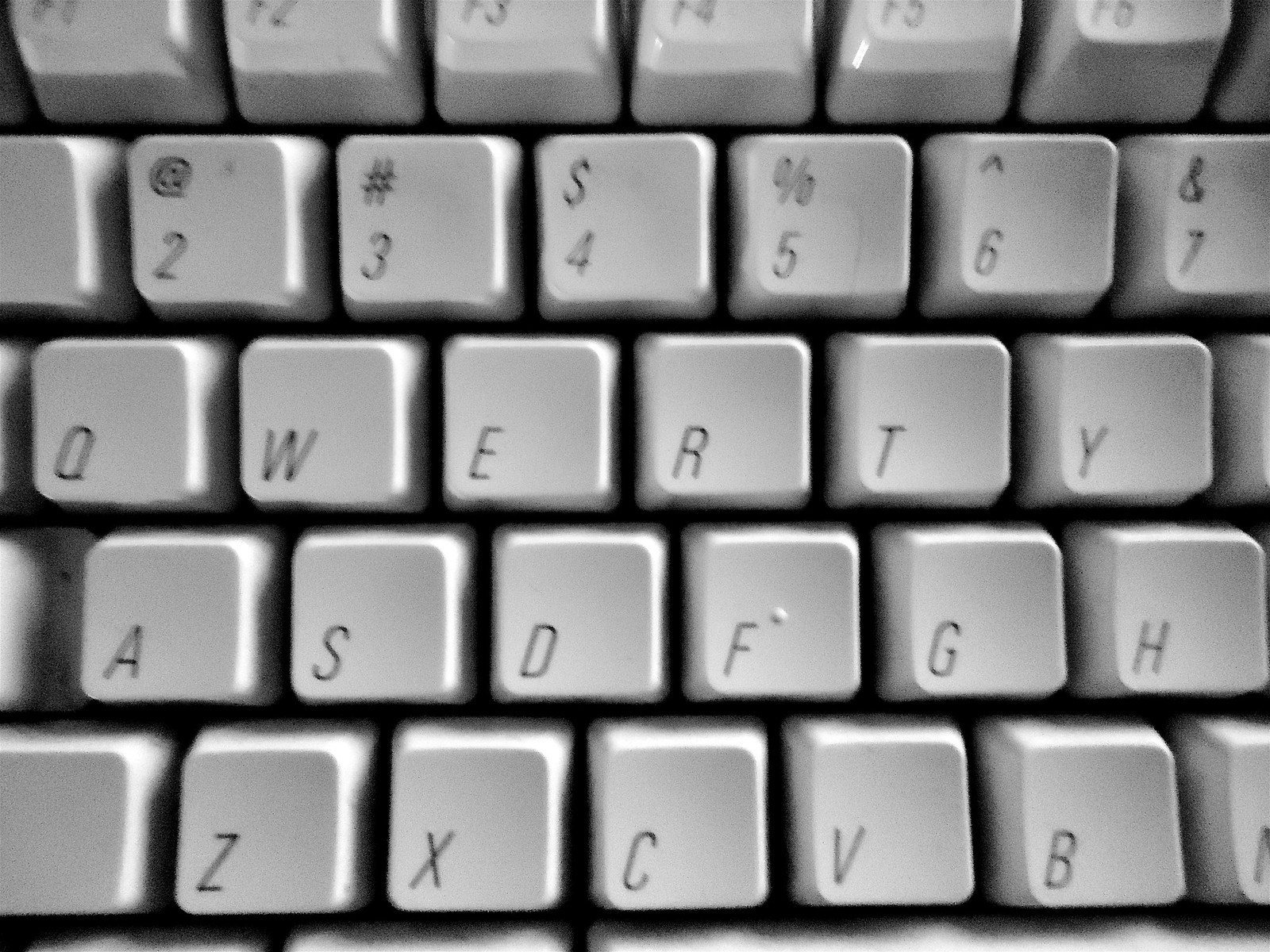This image is a grainy, black and white macro photograph showcasing a vintage or older-style keyboard with raised keys. The focal point is a close-up of white or light-colored keys, detailing their italicized capital letters, numbers, and symbols. The keyboard layout is partially visible, from the bottom-left showing the letters "Z, X, C, V, B," followed by the row above featuring "A, S, D, F, G, H," then "Q, W, E, R, T, Y" and a partially cut-off top row displaying numbers and function keys, including "2 with @, 3 with #, 4 with $, 5 with %, 6 with ^" and so on. Each key has black lettering in the lower left-hand corner. The photograph captures the dark shadows and spacing between the keys, with light, varying shades of gray from the lighting creating shadows along the edges of the square keys and beneath them.